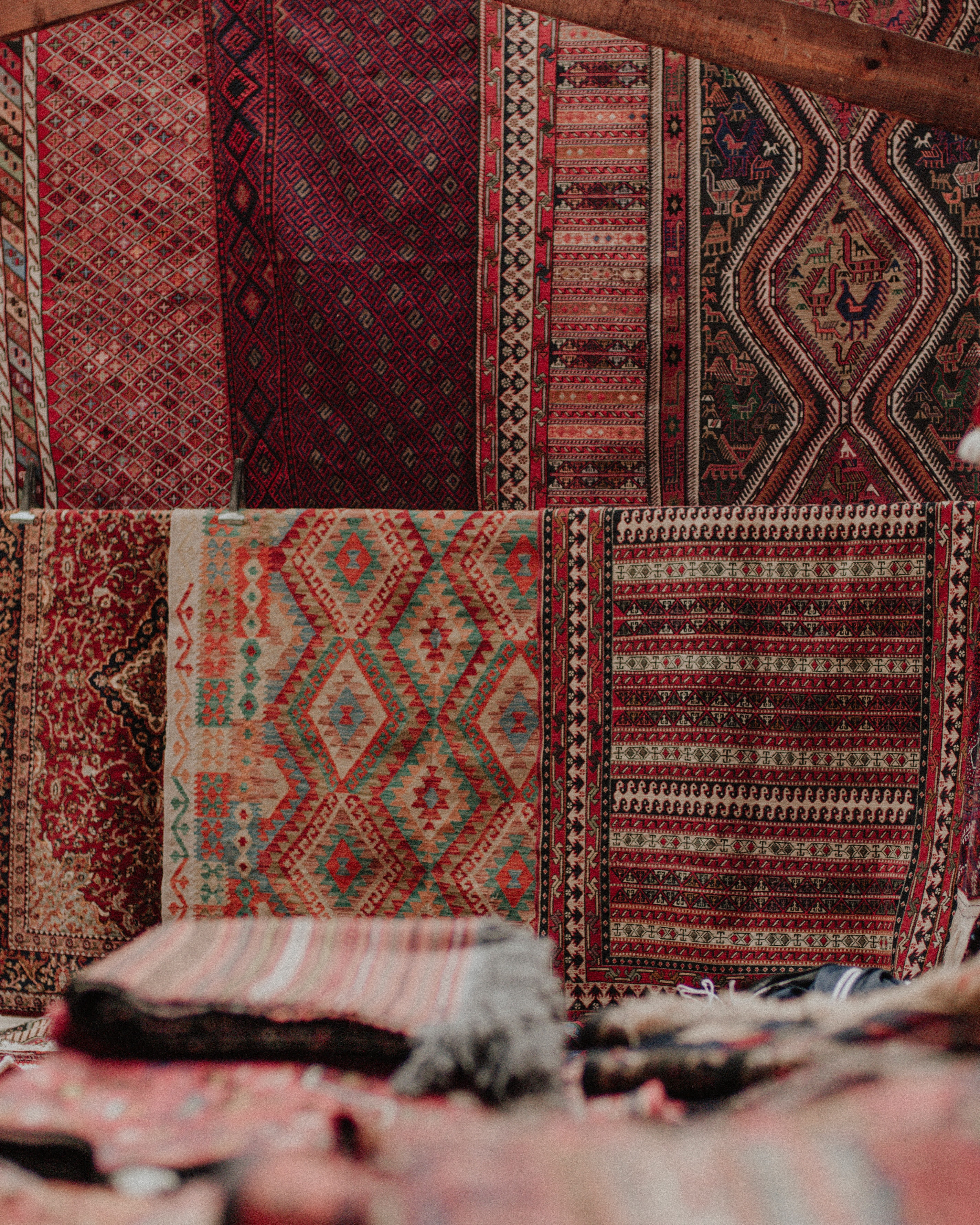The photograph captures a vibrant display of intricately patterned fabric, with a dominant presence of red hues complemented by black, white, gray, green, teal, light blue, and occasional orange. These fabrics, potentially used for rugs, tapestries, quilts, or clothing, are hung for easy viewing, revealing clusters of diamond shapes and other geometric patterns. Notably, some designs include non-geometric shapes like images of chickens. The fabrics are arranged on a wire, overlapping in three distinct sections, with additional longer pieces hung higher, framed by wooden beams visible in the top corners of the image. Below this colorful display, folded linens or rugs are stacked, though slightly blurred, suggesting an artisanal showcase, possibly for sale. The absence of text or identifiable individuals leaves the function of the fabrics open to interpretation.